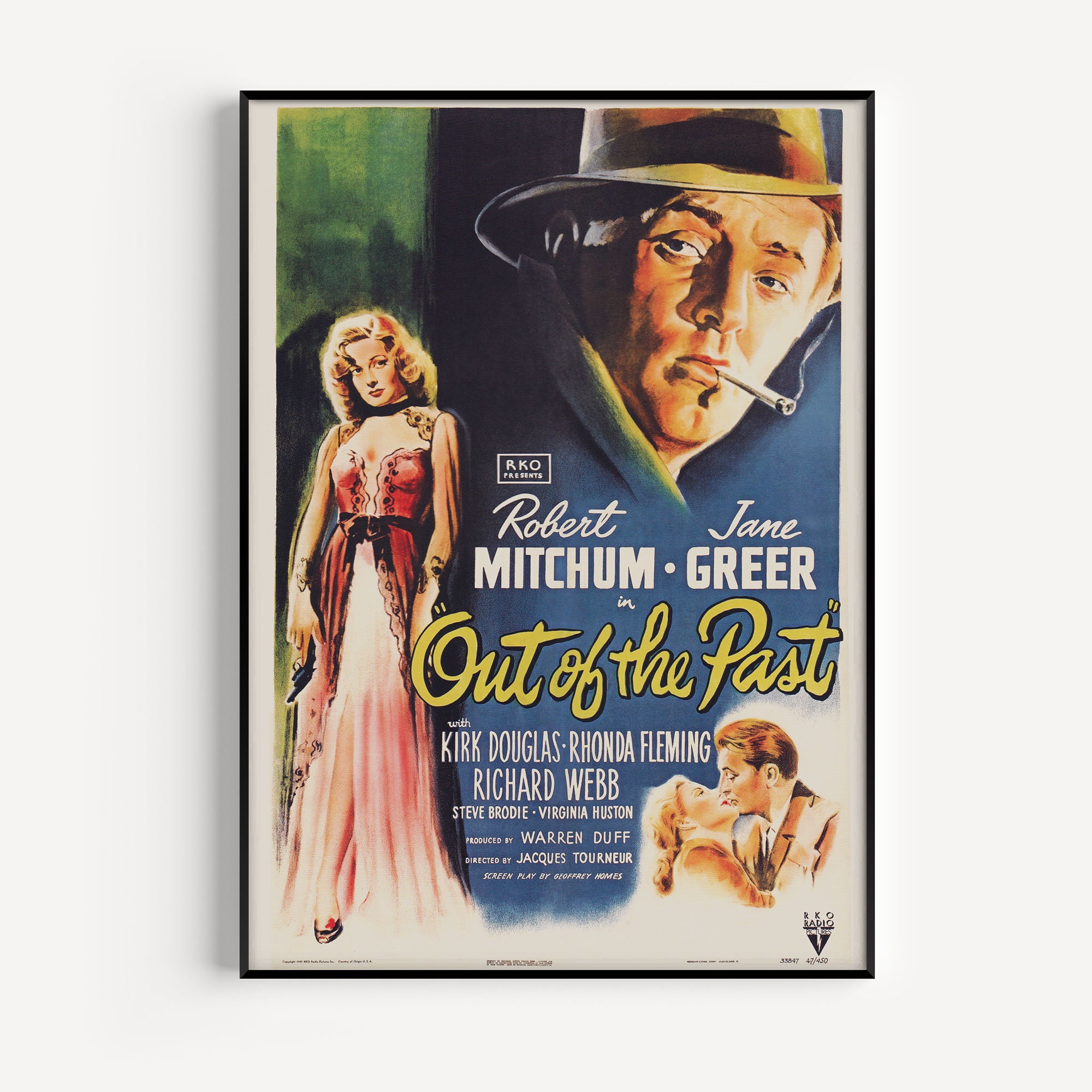The framed poster promotes the classic film "Out of the Past" and is styled with a distinct comic book flavor. The backdrop is white, contrasted by a black thin-bordered frame. The movie title, "Out of the Past," is prominently displayed in yellow cursive writing. Above the title, it reads "RKO presents Robert Mitchum" and "Jane Greer," with their first names in cursive and last names in all caps. Additional cast members, including Kirk Douglas, Rhonda Fleming, and Richard Webb, are listed below in white text. The poster also credits Warren Duff as the producer and Jack Tournier as the director.

The upper right corner features an illustrated image of Robert Mitchum's character, depicted with a fedora hat and a cigarette dangling from his mouth, glancing to the left. He wears a parka coat with a brimmed hat that has a ribbon. The lower left showcases Jane Greer's character in a sultry red dress with a black collar ribbon and a black sash around her waist, holding a black gun. In the bottom right, there is a romantic image of Robert Mitchum and Jane Greer embracing and kissing. The overall appearance suggests an older film, with a faded, vintage feel to the design.